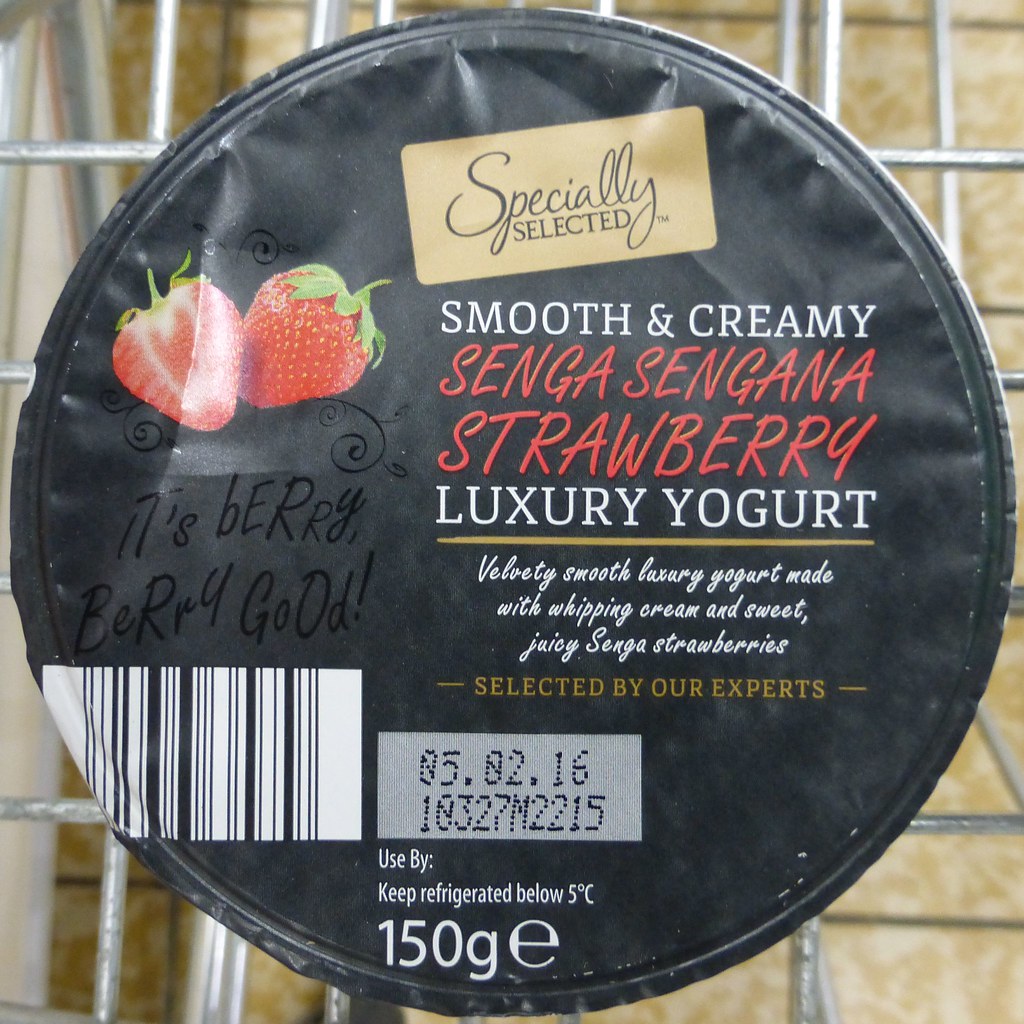This image showcases the top label of a "Specially Selected Smooth & Creamy Senga Sengana Strawberry Luxury Yogurt" container. The photograph appears to have been taken from above, possibly inside a shopping cart, as evidenced by the visible metal bars and the yellowish flooring beneath. The yogurt's circular label, predominantly black, features a vibrant image of two realistic strawberries on the left.

Central to the design, the luxurious branding is emphasized with the text "Specially Selected" in a rounded rectangle, followed by "Smooth & Creamy" and "Senga Sengana Strawberry Luxury Yogurt" in elegant fonts. Directly beneath, it reads, "Velvety Smooth Luxury Yogurt Made With Whipping Cream & Sweet Juicy Senga Strawberries Selected By Our Experts." A bronze-colored text highlights the expert selection of the strawberries.

Additional details include the expiration date, "5-2016" and a code "103-27N-2215." The label also notes "Keep Refrigerated Below 5 Degrees Celsius", and that the container holds "150 Grams" of yogurt, marked with an 'e'. A UPC barcode is located towards the bottom left, with the phrase "Berry Berry Good" inscribed below it.